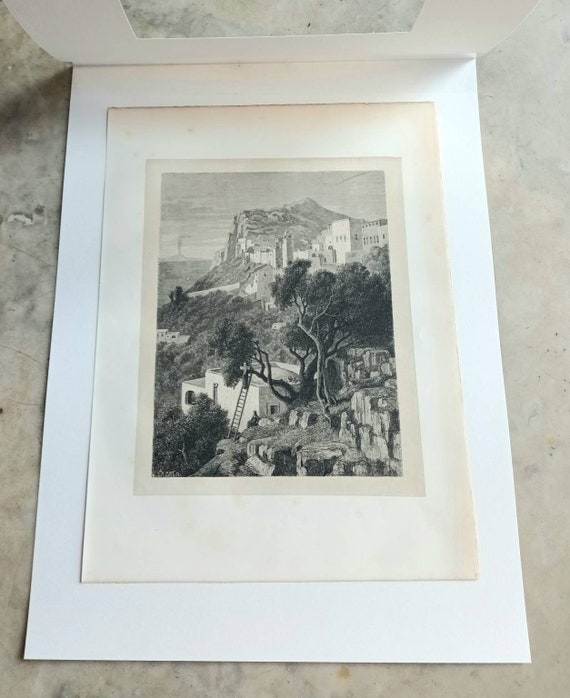On a polished granite countertop lies a weathered photo envelope made of durable cardstock, which opens to reveal a black and white drawing or photograph. The drawing depicts a picturesque, Mediterranean-like village perched on a cliff, with boxy, adobe-styled, or stucco houses scattered among scrubby trees and rocky outcroppings. In the background, a smoking volcano adds a dramatic backdrop to the serene setting. Among the houses, a ladder leans against one structure, where a man appears, his form somewhat cruciform. The artwork, somewhat aged with a yellowed hue, is mounted on a fresh white matting that contrasts with the older paper. This setup, though, gives the drawing the effect of almost being hinged by the matting, which when folded down, would frame the picturesque scene. The entire arrangement sits against the granite surface, enhancing the timeless beauty of the captured moment.